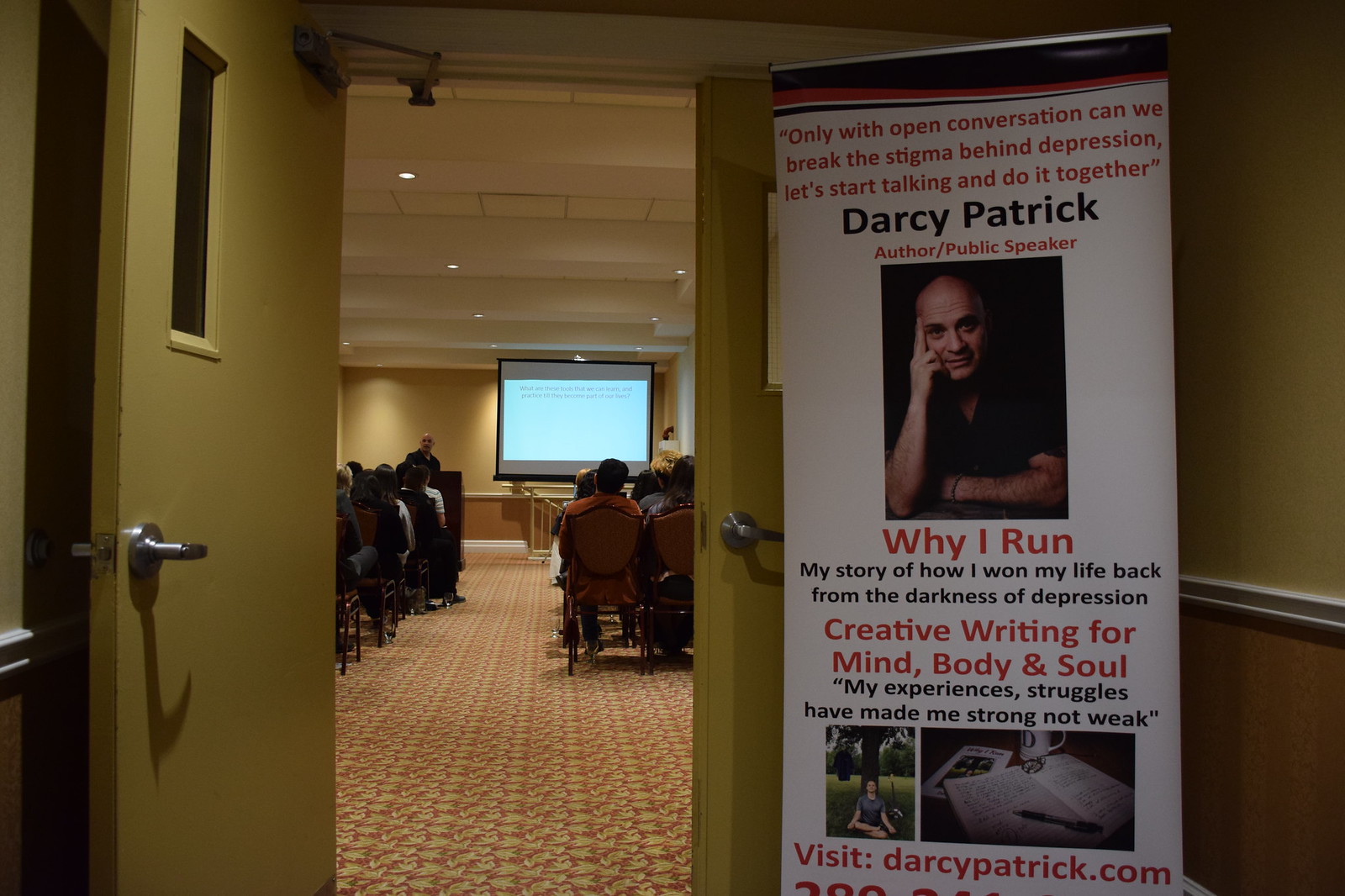The photograph captures the entrance to a small, hotel conference room currently serving as an auditorium. The open left door, part of a set of yellow-green doors, reveals a crowded audience seated in rows of chairs facing a speaker at a podium. The speaker, identified as Darcy Patrick—an author and public speaker—is delivering a lecture focused on breaking the stigma surrounding depression, as indicated by a tall white banner to the right of the entrance. The banner reads, "Only with open conversation can we break the stigma behind depression. Let's start talking and do it together," and features a photo of Darcy Patrick along with additional text. Inside, a large projector screen on the left side of the room displays slides related to the talk. The ceiling is adorned with small white lights, while the room's walls are painted yellow and the patterned flooring incorporates red, white, and yellow elements.